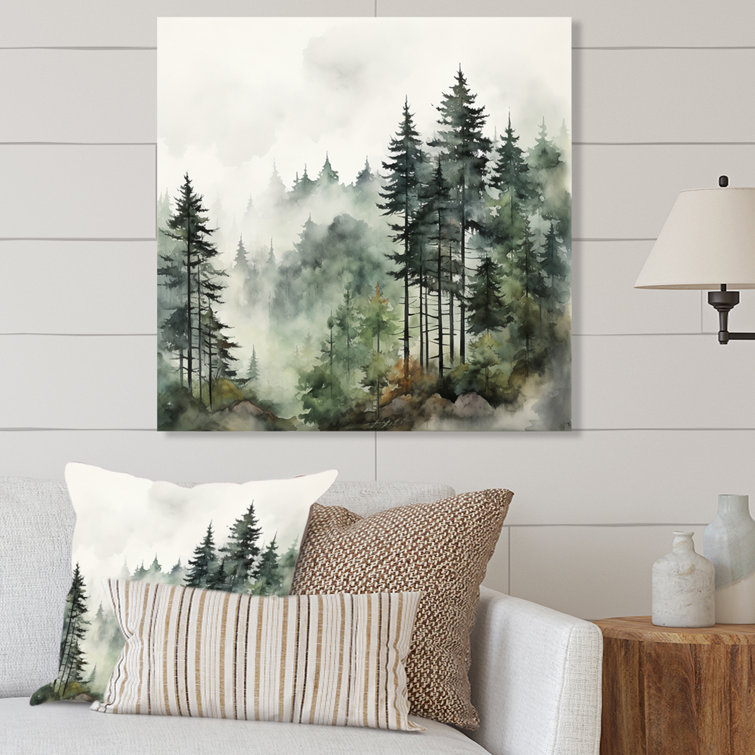This indoor color photograph captures a close-up view of a cozy living room corner. The focal point is a square painting on the white paneled wall, depicting a fog-laden mountain scene with towering conifer trees, their tall trunks rising prominently amidst a misty, clouded background. Directly beneath the painting is an off-white couch adorned with several cushions: one featuring artwork akin to the painting, a plain white pillow, a brown pillow, and a striped brown and gold pillow. To the right of the couch stands a small wooden side table, rustic in appearance, bearing two empty ceramic vases with a marble-like finish. A floor lamp with a white shade and a black handle peeks into the scene from the upper right corner, subtly illuminating the serene, woodland-themed decor.